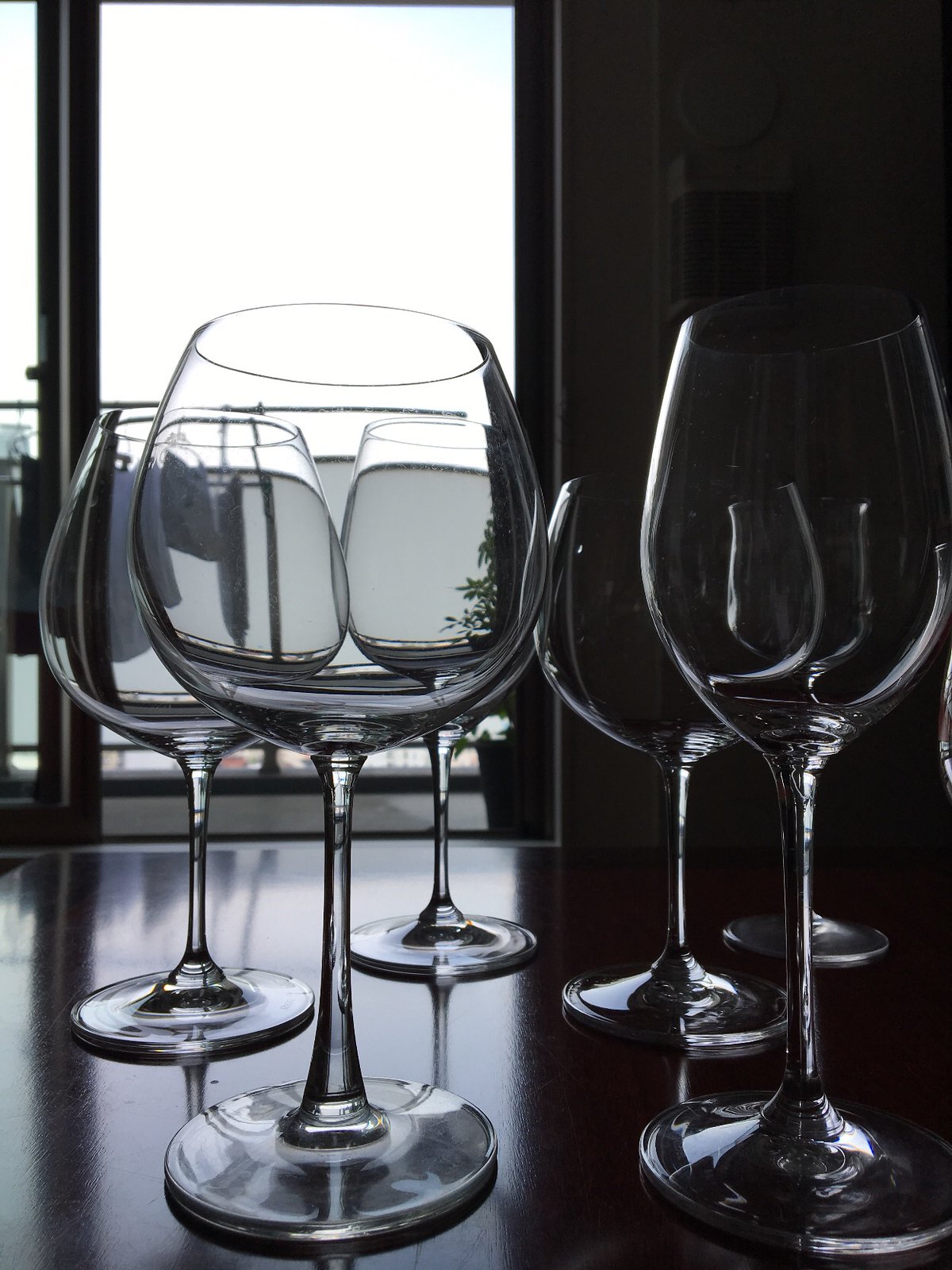This photograph captures a dimly lit indoor scene, predominantly in black and white, emphasizing shadows and low light. The focal point is a dark, shiny table or bar where six different types of empty wine glasses are meticulously arranged. Some are narrow while others have wider bowls, showcasing a variety of wine glass styles. Behind the glasses, a window filters in scant, dim sunlight, creating subtle reflections on the table's surface and casting intricate shadows. The light also produces a faint, distorted view through the glasses, hinting at a railing and possibly a bush outside. The window frame and nearby walls are dark, deepening the shadowy atmosphere of the scene. The meticulously composed arrangement of the glasses, their reflective surfaces, and the interplay of light and shadows craft a visually arresting and detailed image.